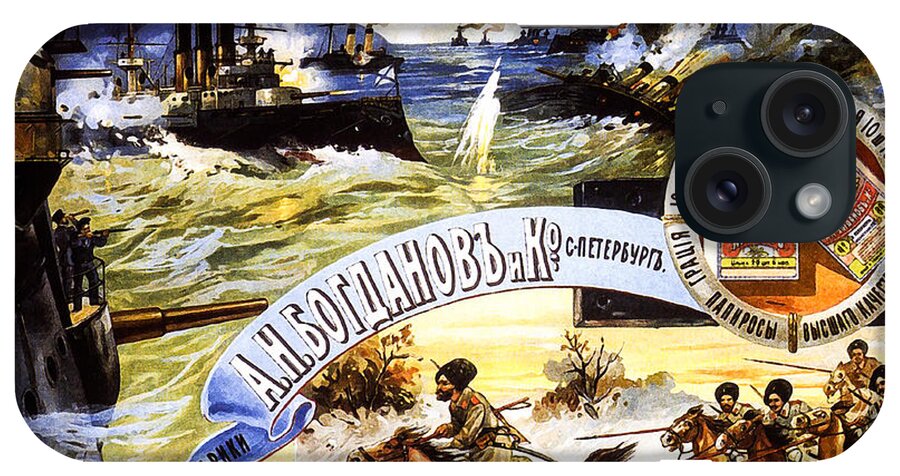This image is a detailed and vibrant historical painting, seemingly a Russian poster, that vividly portrays a dramatic battle scene both on land and sea. In the foreground, a group of Cossack cavalry charges forward through shallow water, brandishing lances, swords, and an archer with a bow slung across his back. They are distinguished by their traditional attire, including turbans and bearskin caps. The background showcases a fierce naval battle, with steamships racing towards the shore, cannons firing, and the water splashing yellow from the impacts of cannon shots. On the left side, sailors can be seen on a battleship, manning the cannons and shooting rifles. A large, partially readable white lettering in Russian spans across the image, adding to its historical context. The scene is topped off by a darker colored sky, possibly indicating the intensity and gravity of the conflict depicted.